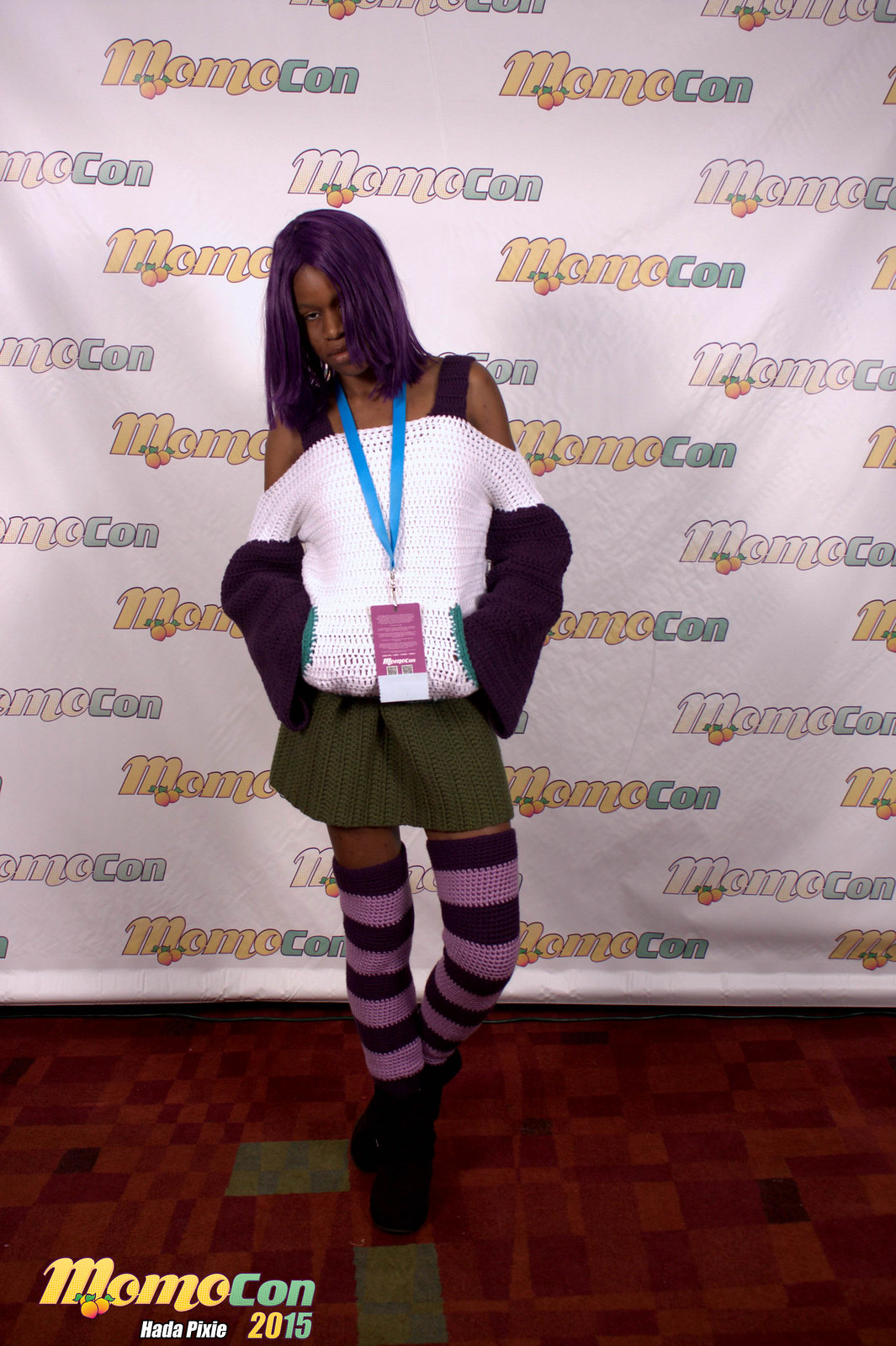The photograph showcases a young African American woman standing against a white backdrop emblazoned repeatedly with the MomoCon logo, which features "Momo" in yellow and "Con" in green, with peaches adorning the letter "M." The woman appears to be around 18 years old and is dressed in a knitted ensemble: a white knit top with long black sleeves, a brown knitted skirt, and thigh-high striped socks in black and gray. She completes her outfit with black shoes. Her long hair, with a purplish hue, falls to her shoulders and is parted to the side. She also wears a bright turquoise lanyard with a rectangular pass hanging from it. The bottom left corner of the image features the text "MomoCon Hada Pixie 2015." The scene is set on a burgundy carpeting with checkered patterns, resembling a red carpet event.